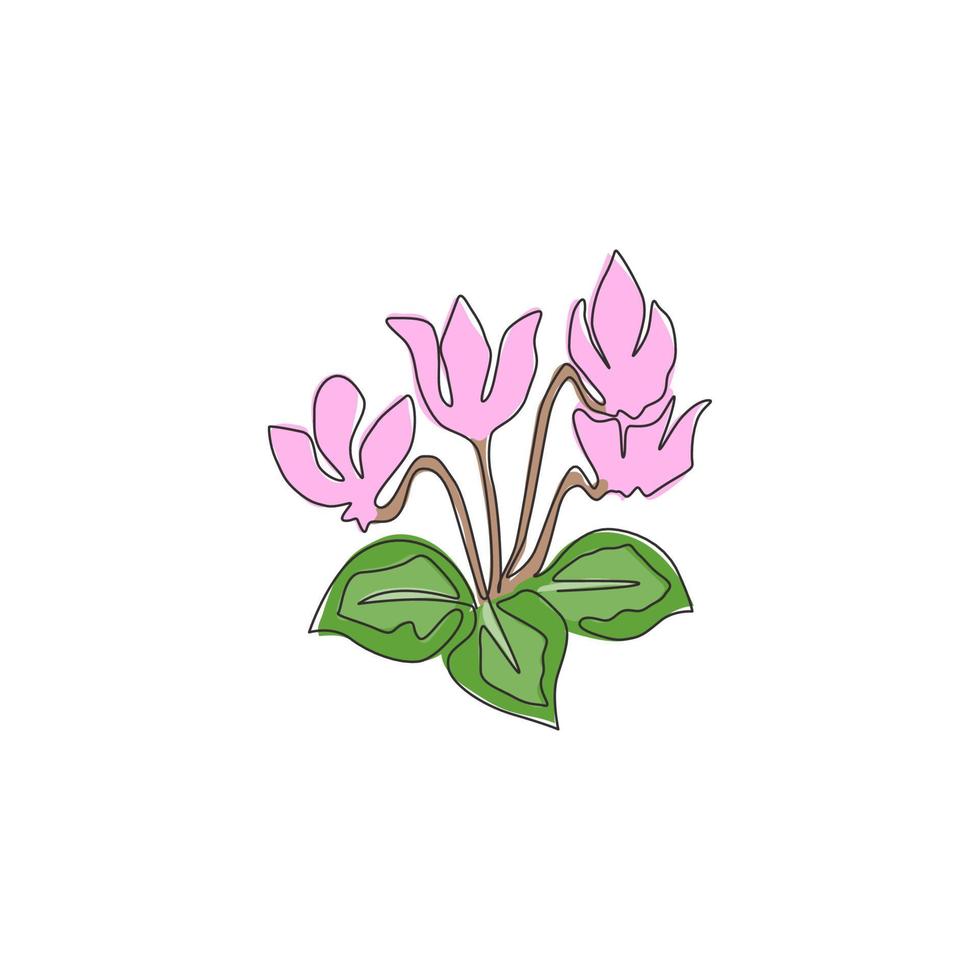The image features a whimsical, amateur-style clipart illustration of a plant against a white background. The drawing appears to have been created with Microsoft Paint or a similar program. The plant consists of four tulip-shaped flowers at the top, each with three light pink petals outlined in black. The pink coloring spills outside the lines and does not completely fill the petal shapes. The stems of the flowers are brown and similarly colored carelessly, with gaps inside the outline. Below the blooms are three teardrop-shaped leaves, each outlined in a darker green with a lighter green interior and a faint central vein. The leaves also have portions where the color extends beyond the black outlines, giving the entire drawing a childlike scribbled appearance.